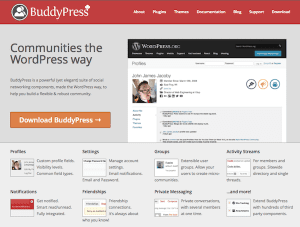This small, highly compressed image is a screenshot under the heading "Websites". At the top of the image, a red line spans horizontally. Prominently displayed are the large, bold letters spelling "BuddyPress". Below this, a circular icon features a white rim and green background, depicting two figures standing back-to-back.

The image also contains several headings near the top, though they are unclear and difficult to decipher, with "Home" being the only semi-recognizable word. Beneath these headings is a gray section featuring the tagline "Communities the WordPress Way", followed by a paragraph of informational text that is not legible in the small image.

Further down, an orange button with white text invites users to "Download BuddyPress", accompanied by an arrow indicating the download action. On the side, a black bar at the top labels a section titled "WordPress". Inside this section is a picture of a man. At the bottom of the image, there are various small boxes, too pixelated to read clearly, though one appears to say "Settings" and another "Storage". The content and details of other boxes remain indiscernible due to the image's compressed nature.